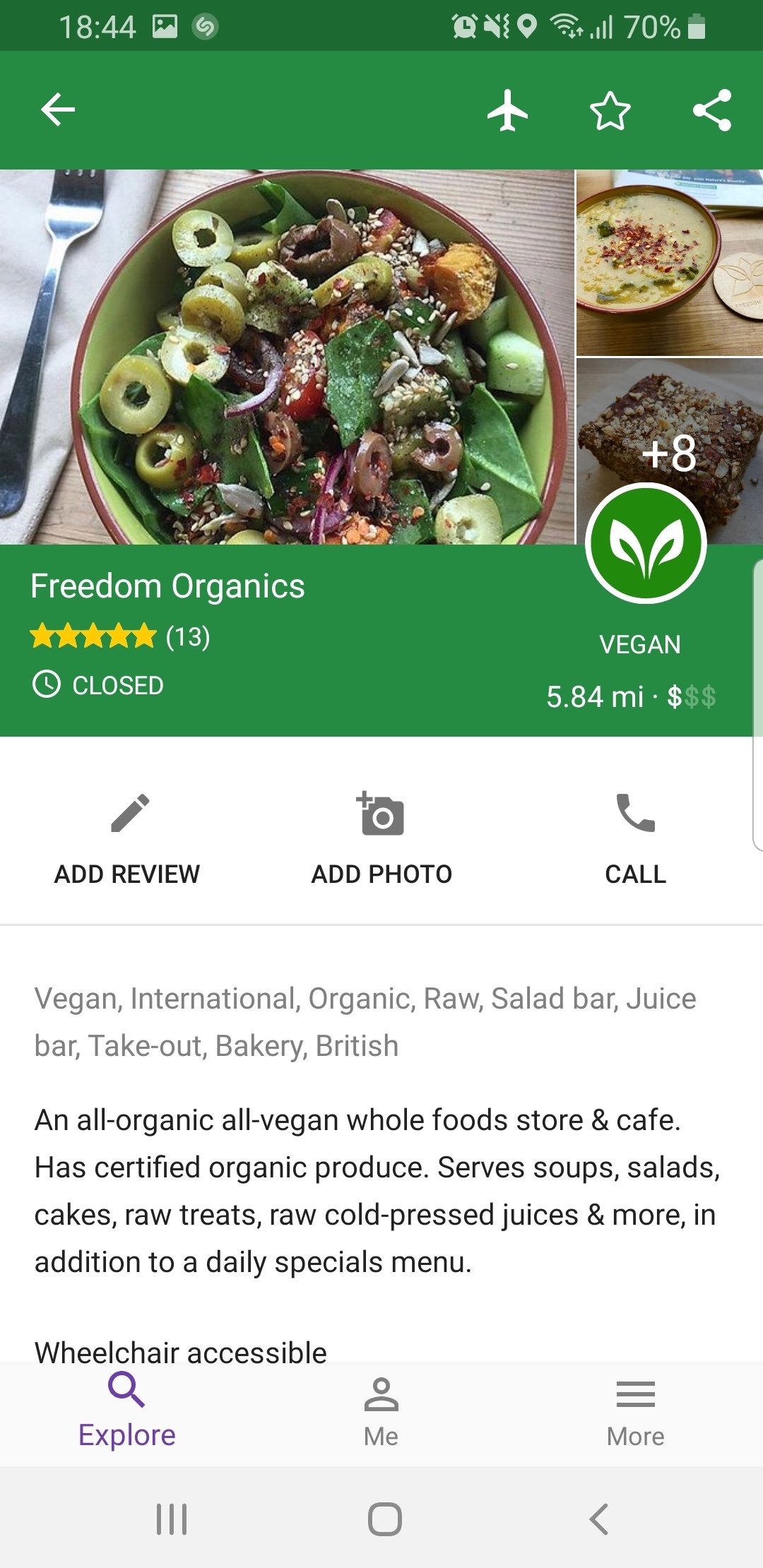This screenshot from Google Maps shows a detailed pop-up of a restaurant called "Freedom Organics." The pop-up includes an image of a vibrant salad bowl featuring olives and fresh leafy greens, indicative of the restaurant's menu offerings. Freedom Organics boasts an impressive 5-star rating based on 13 reviews. The restaurant is celebrated for its vegan, raw, and organic cuisine.

Located 5.84 miles from the user, Freedom Organics isn't considered overly expensive. It features a comprehensive selection including a salad bar, juice bar, and take-out menu, along with bakery items. The restaurant showcases an array of British-inspired vegan dishes, emphasizing all-organic, all-vegan whole foods. Additionally, the establishment has certified organic produce and offers an extensive menu that includes soups, salads, cakes, raw treats, and cold-pressed juices. Various user-uploaded images also accompany the pop-up, providing further visual insight into the restaurant’s offerings and atmosphere.